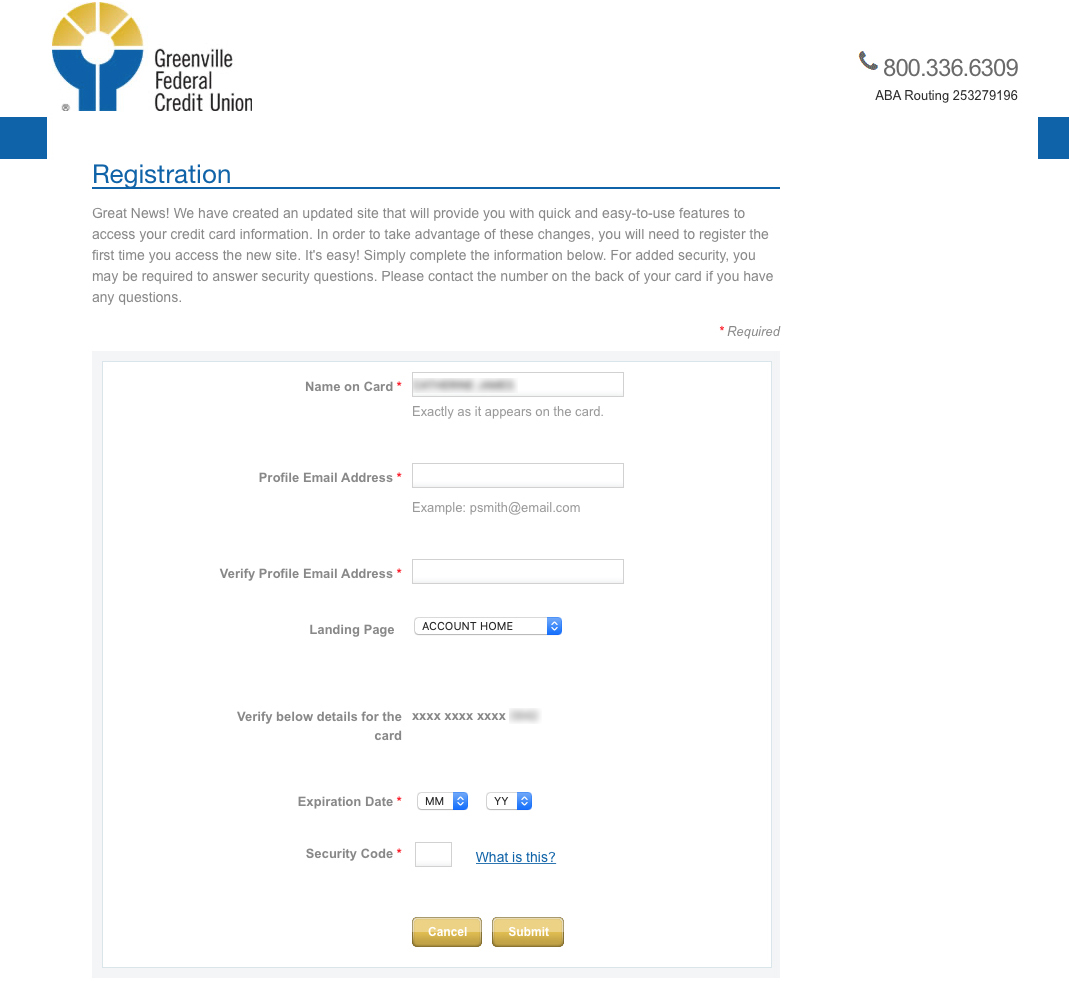The image depicts the newly updated Greenville Federal Credit Union website. On the left side of the screen, the Greenville Federal Credit Union logo is prominently displayed. It features a round head-like shape with blue arcs extending upward on either side. The upper portion of the logo contains four sections of yellow and a blue square to the left.

Adjacent to the logo, the website prominently displays a 1-800 customer service number and the ABA routing number for user convenience. There is also a small blue rectangle, which might be a button or an indicator.

The main section of the page announces, "Great news! We have created an updated site that will provide you with quick and easy-to-use features to access your credit card information." To access these new features, users are required to register by completing the form provided.

The registration form includes:
- Name on card (required), exactly as it appears on the card.
- Profile email address (required).
- Verification of the profile email address (required).
- A selection field for the landing page with "Account Home" as an option.
- Verification of additional details, including an example card number.
- Expiration date in months and years (available as dropdown menus).
- Security code (CVV), with an informational prompt labeled "What's this?"

Finally, two gold buttons at the bottom of the form allow users to either "Cancel" or "Submit" their registration information. 

Instructions advise that, for added security, users might be required to answer security questions. If any help is needed, users are encouraged to contact the number on the back of their card. Fields marked with a red asterisk (*) indicate required information.